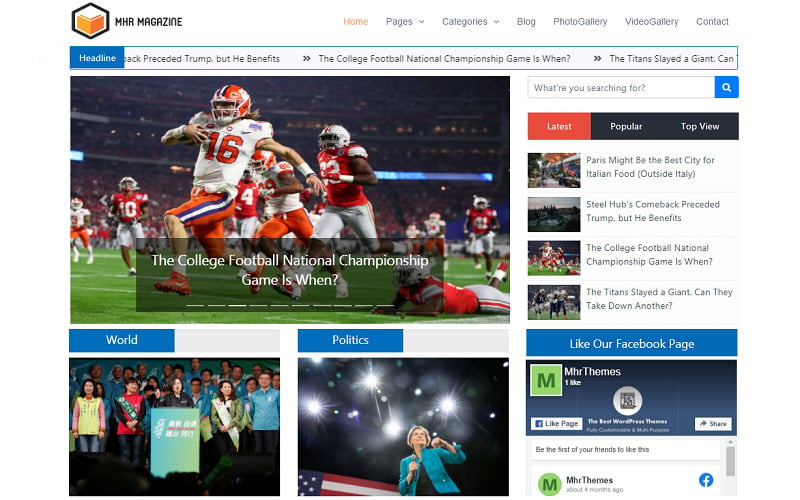This is an image displaying a web page from "MHR Magazine." The web page header features a block colored in vibrant orange, bordered by a three-dimensional black outline. This is prominently designed to catch the eye. 

Just below the header, there is an orange "Home" button. In black text, there are additional navigation options labeled as "Pages," "Categories," "Blog," "Photo Gallery," "Video Gallery," and "Contact."

At the top of the page, a blue headline is partially visible, stating "Back Preceded Trump, But He Benefits." However, the first part of this headline is cut off. Beneath this, another headline asks, "The College Football National Championship Game is When?" Nearby, there are arrows suggesting more articles, one of which mentions, "The Titans Slayed a Giant Can," though this headline is truncated.

Scrolling down reveals several articles. One prominently featured article repeats the headline, "The College Football National Championship Game is When?" showcasing an image of football players, presumably from Georgia and Ohio State, in action.

In the background, there are sections marked "World" and "Politics." Additional features include prompts to "Like Our Facebook Page," and labeled tabs in red for "Latest," "Popular," and "Top View" articles, helping visitors quickly find trending content.